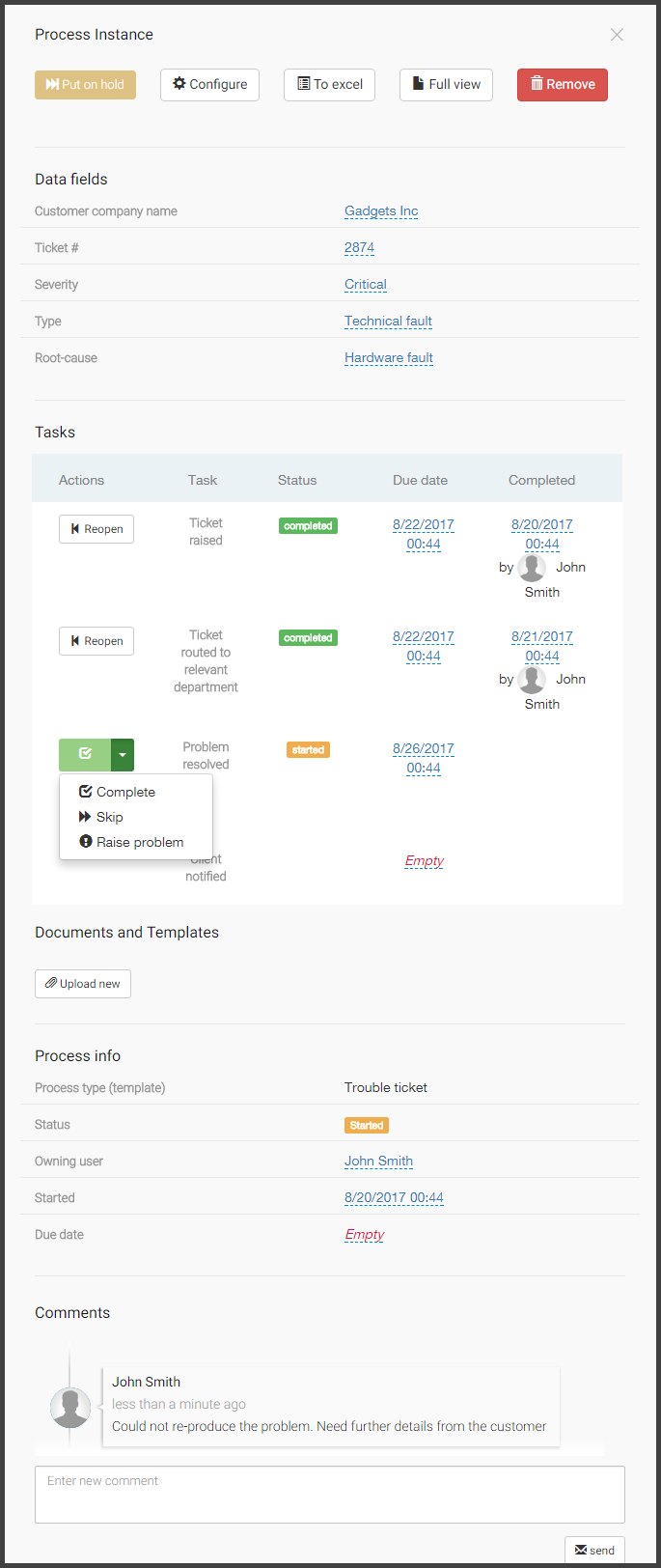The image depicts a help desk interface showing the details of a trouble ticket. The header reads "GadgetSync Ticket 2874" with the severity marked as "Critical" and the type classified as a "Technical Fault" due to "Hardware Fault."

Below the header, the "Data Fields" section outlines relevant information:
- Customer Company Name:
- Ticket Number: 2874
- Severity: Critical
- Type: Technical Fault
- Root Cause: Hardware Fault

A "Complaint Ticket Review" section details the ongoing actions and status:
- Tasks:
  1. Action: Reopened Ticket | Status: Completed | Due Date: 08/20/2017 | Completed By: John Smith
  2. Action: Ticket Routed to Relevant Department | Status: Completed | Due Date: 08/21/2017 | Completed By: John Smith
  3. Action: Complaint Resolved | Status: Completed | Due Date: 08/22/2017 | Completed By: John Smith

The interface features drop-down options labeled "Complete," "Skip," "Raise Problem," and "Problem Resolved," among others.

At the bottom, there are fields and options for "Templates and Documents" with buttons for "Upload," "View," and "Process Info." The "Process Type" is noted as "Trouble Ticket" with the status "Started," owned by "John Smith," initiated on 08/20/2017 at 00:44. The due date remains unspecified. 

Comments section:
- Comment by John Smith (less than one minute ago): "Could not reproduce the problem. Need further details from the customer."

An "Enter New Comment" field is available for additional input.